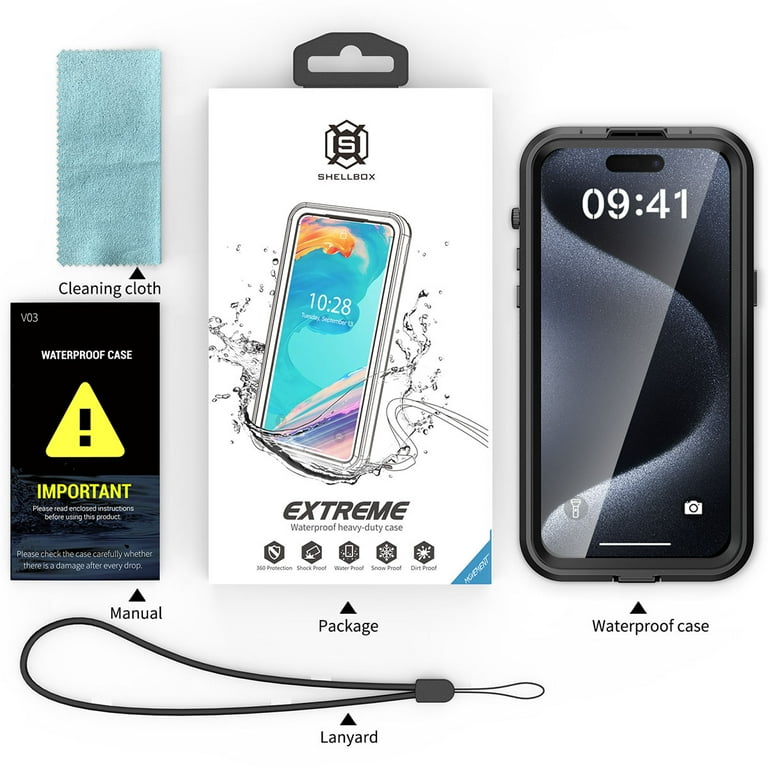This image depicts a retail package for a waterproof, heavy-duty phone case from the brand "Shell Box." The front of the box prominently features the word "EXTREME" and includes the product description. The Shell Box logo, represented by an "S," is displayed at the top. The packaging is designed for retail display, with a clip attached for hanging on store racks.

To the right of the box, several items are showcased to highlight the product's contents and features. These include a smartphone encased in the waterproof cover, displaying the time "9:41" on the screen. Along the bottom of the image, a lanyard is neatly arranged, showcasing an additional accessory included with the waterproof case.

Also featured is an image of the user manual, marked with an important warning symbol to ensure users recognize its significance. Lastly, a blue cleaning cloth is included, emphasizing the package's comprehensive nature in providing both protective and maintenance tools for the phone case.